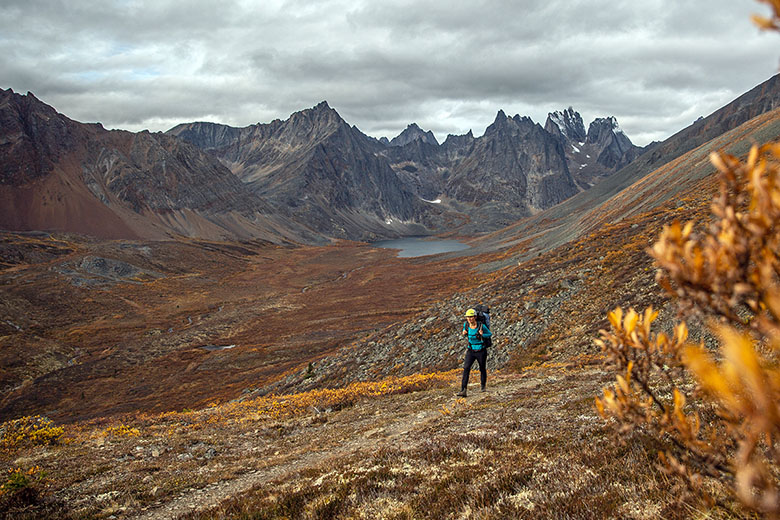In this color photograph, a woman is seen hiking through a barren wilderness in the mountains on an overcast day, under heavy, gray clouds. She is wearing hiking boots, black leggings, a bright blue shirt, and a yellow helmet or hat. She carries a substantial backpack that appears to be black and possibly blue. The rocky mountains in the background are craggy and devoid of vegetation. A small lake is visible in the valley far off in the distance. The foreground features a brownish-orange plant with golden leaves and a few scattered flowers. Despite the minimal sunlight, the scene is vivid with a few patches of grass and some snow evident on the mountain tops. The hiker, captured in motion, appears diminutive against the vast and rugged mountain landscape, walking towards the left bottom corner of the photograph.